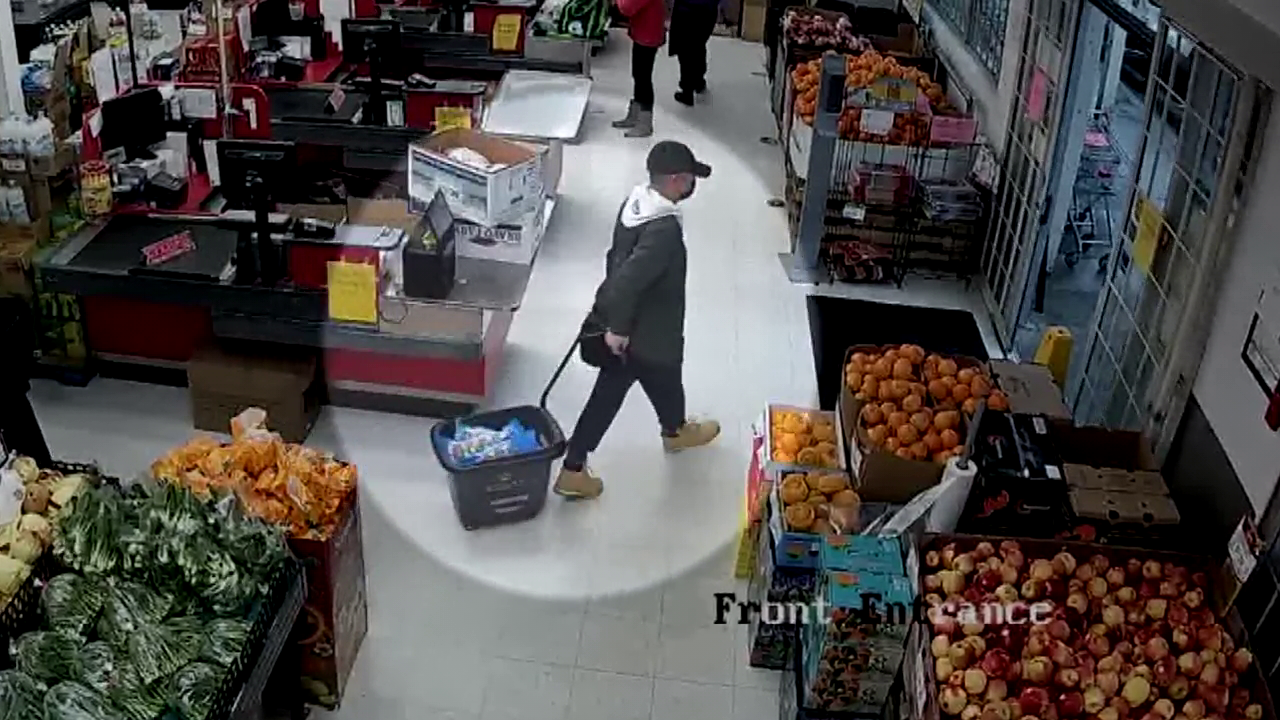This detailed color photograph, likely taken from a security camera, captures the front checkout lanes of a bustling grocery store. The checkout lanes, painted in red and black, feature conveyor belts ready for customer use. The store's front entrance is visible, with open exit doors hinting at the activity within. In the foreground and lower corners of the image, numerous boxes overflowing with fresh produce such as apples, oranges, and various green vegetables are neatly arranged.

However, the focal point of the image is a particular individual highlighted by a white circle. This person, dressed in a gray hoodie, dark pants, and brown boots, is seen carefully pulling a rollable shopping basket filled with food. The man also sports a gray baseball cap that partially shades his forehead and eyes. There are additional people in the background, although their faces are partially obscured. The emphasis on the highlighted man suggests he is of particular interest, perhaps to security, given the context of the image.